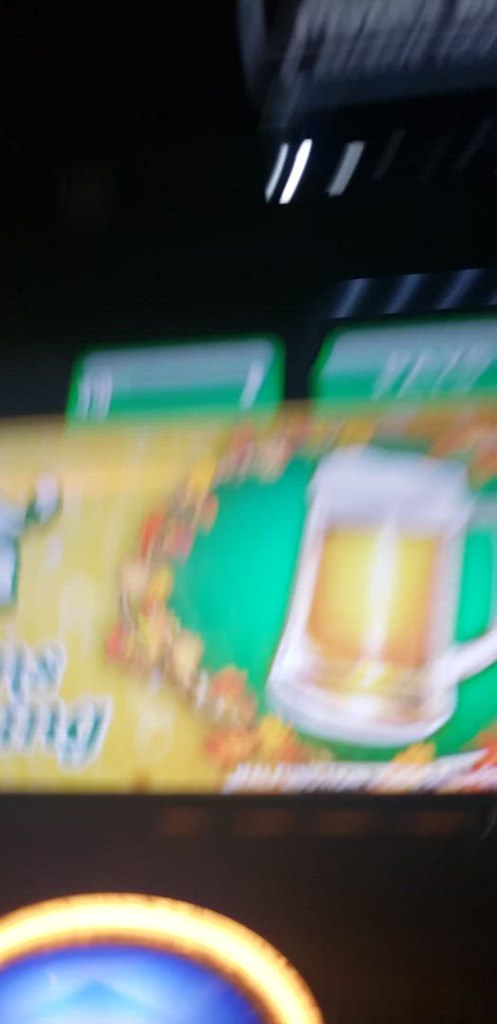The blurred image appears to be a photograph of a sign or billboard. The main focus is a white-handled beer mug with an orange or brown beverage inside, topped with white froth. This mug is set against a green background, encircled by a pattern of yellow and orange autumn leaves. To the left, inside a yellow section, there is some blue text, although only the letters "ING" are discernible. Above this section are two green rectangles with faint white lines running vertically. At the lower left corner, there's a semi-circle filled with bright blue, outlined by an orange ring. The overall scene seems out-of-focus but suggests a vibrant and somewhat intricate design.